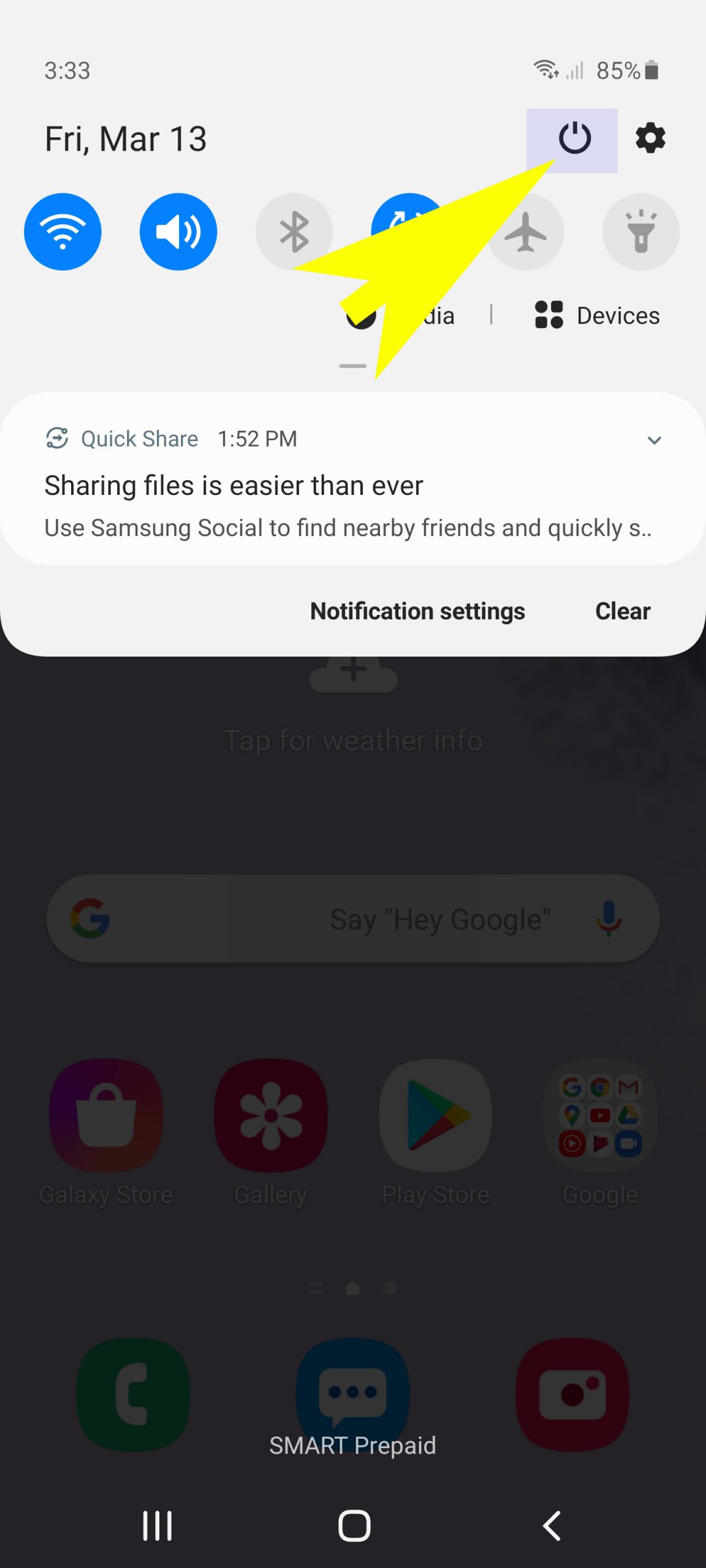In this cell phone screenshot, the time displayed at the top left corner is 3:33 PM. On the top right, the Wi-Fi signal is at full strength, the cell phone signal is nearly empty, and the battery level is at 85%. The date indicated is Friday, March 13th. Adjacent to the date on the right side, there are power and settings buttons. A large, hand-drawn yellow arrow is pointing towards the power button.

Beneath this, a row of icons is visible: the first icon shows the Wi-Fi signal strength, the second indicates volume control, the third is for Bluetooth, the fourth icon (obscured by the yellow arrow) is unreadable, the fifth icon is for airplane mode, and the sixth is a flashlight icon. The Wi-Fi, volume, and the partially obscured icon are highlighted in blue with white symbols.

Below the icon row is a drop-down box labeled "Quick Share" at 1:52 PM with further icons and options to manage sharing. The text beneath it reads: "Sharing files is easier than ever using Samsung Social to find nearby friends and quickly," and the rest is cut off. Below this, there are options for "Notifications" and "Clear."

The background behind this presented information is split into two sections: the top half is white, and the bottom half is grayed out. This grayed-out section appears to be an effect of the active Quick Share button. In the grayed-out section, several app icons are semi-visible including the Google Search bar, Google Play Store, a gallery app, Galaxy Store, and a Google folder with nine icons. At the bottom, the home screen shows docked icons for phone, chat, and camera functions. The text "Smart Prepaid" is visible in white, along with three circular navigation buttons—the middle circle for the home screen, and an arrow pointing to the left.